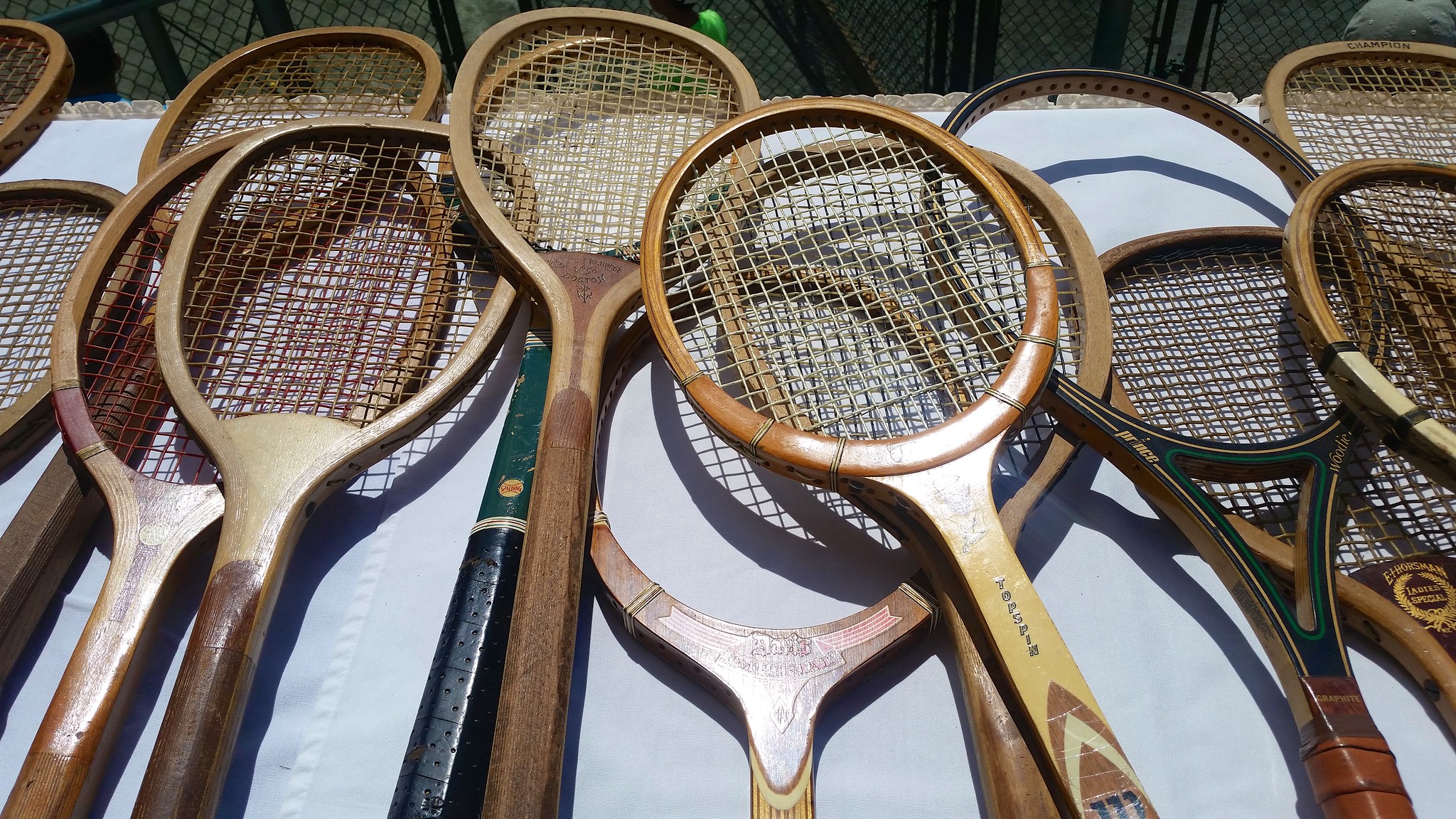The image displays a collection of vintage wooden rackets, each with a wooden handle and frame, spread out across a blue table, some stacked three or four deep. The rackets are predominantly brown, with netting that appears aged. A notable racket features a green and black handle with a small yellow emblem and the name "Top Spin" on it. Another racket with green elements is missing its netting. The table is covered with multiple white tablecloths, visible through their seams. In the background, a dark area reveals a chain-link fence, a green leaf, and the shadows cast by the rackets, adding depth to the scene.